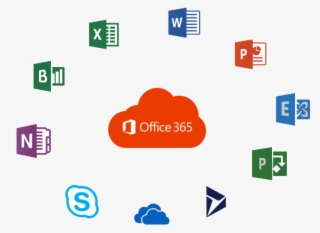The image is an advertisement for Microsoft Office 365, showcasing its suite of applications. It features a four-by-three aspect ratio, slightly wider than it is tall, and has a clean, white (or off-white) background. Central to the design is an orange cloud icon, prominently displaying the "Office 365" text alongside the recognizable Open Book logo in white. Surrounding this centerpiece in a circular formation are the individual icons for various Microsoft Office apps. These include:

- A blue "W" for Word
- An orange "P" for PowerPoint
- A blue "E" for Excel
- A green "P" for Publisher
- An abstract icon composed of two triangles and a quadrangle for Access
- The OneDrive icon, depicted as two cloud shapes
- The Skype icon, featuring an "S" within a semicircular design

The overall layout and iconography highlight the comprehensive range of tools available within the Office 365 suite.